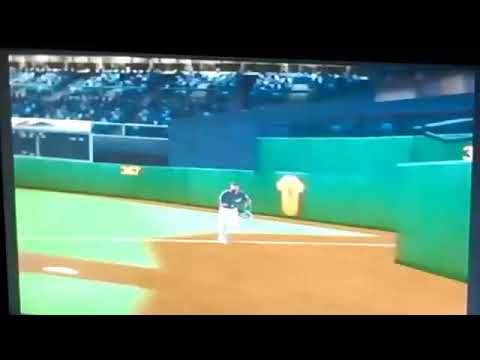This image depicts a heavily stylized, digital photograph of a television screen displaying a scene from a baseball game. The television screen itself is framed by black bars at the top and bottom. At the center of the image is a baseball player with light skin, wearing a blue shirt and white pants, seemingly running to catch a ball, though the ball itself is off-screen. The player stands against a turquoise green outfield wall, with deeper blue, likely empty, stadium seats visible behind the wall. The wall features a conspicuous white outline of a shirt, while the field transitions from light greenish-blue grass on the left to a beige, sand-like surface on the right. The overall image appears blurry and low-resolution, likely resulting from the picture being taken directly off a television screen.